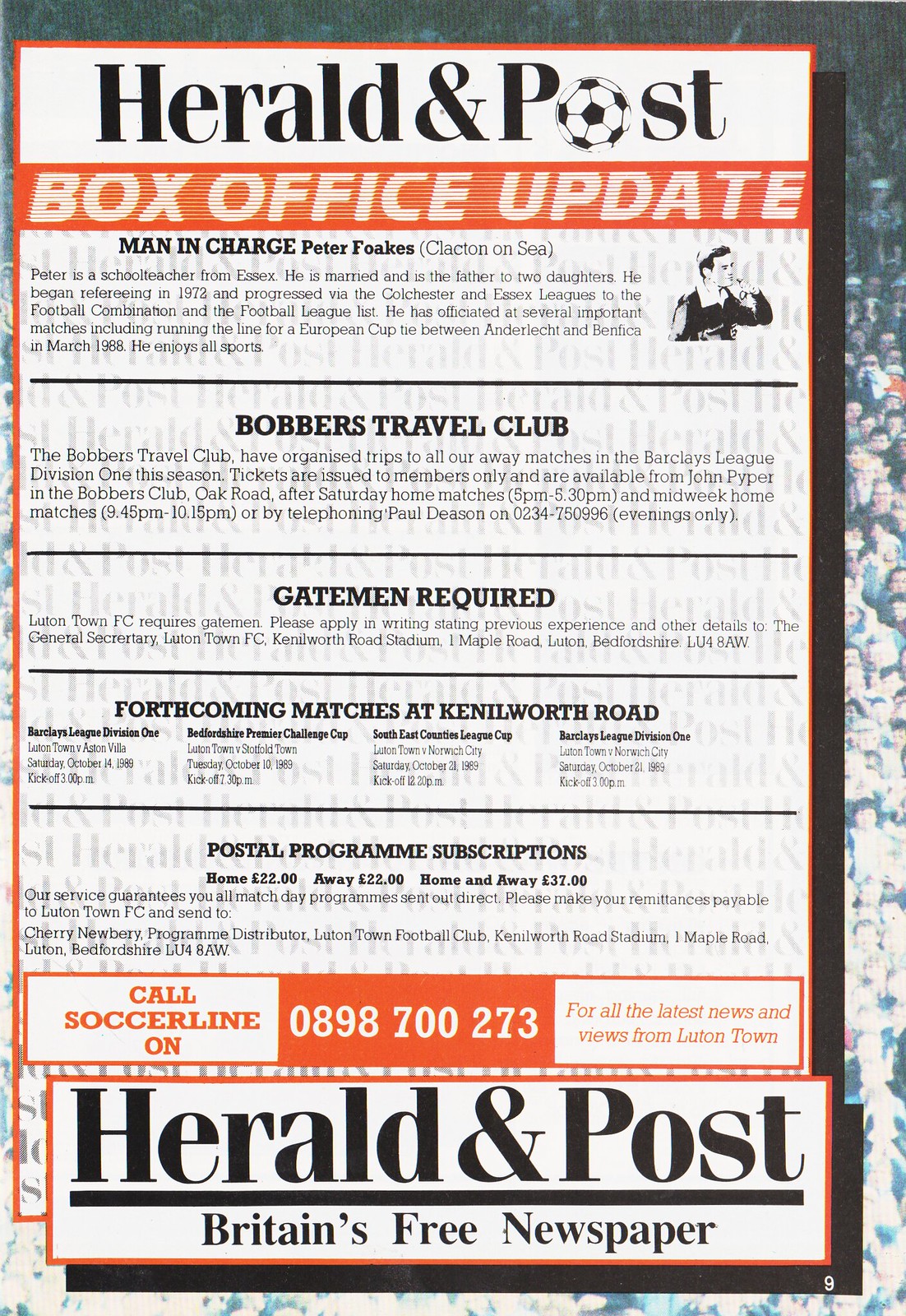The image depicts the portrait-oriented front cover of the Herald and Post, Britain's free newspaper, set against a background photo of a stadium crowd. The cover has a narrow orange outline and features a prominent "Herald and Post" header in black text on a white background, with a soccer ball icon replacing the "O" in "Post." Below this header, an orange strip spans the width of the page, displaying "Box Office Update" in bold white uppercase letters.

The main article, titled "Man in Charge," profiles Peter Folks. Peter is a school teacher from Essex, married with two daughters. He began refereeing in 1972 and progressed through the Colchester and Essex leagues to reach the football combination and the football league list. His impressive career includes officiating significant matches such as a European Cup tie between Anderlecht and Benfica in March 1988. Peter enjoys all sports.

Additional sections on the cover include:

1. "Bobbers Travel Club," detailing organized trips to all away matches in the Barclays League Division 1 this season.
2. "Gateman Required," a notice from Luton Town FC seeking gatekeepers.
3. Forthcoming matches at Kenilworth Road, listing Barclays League Division 1, Bedfordshire Premier Challenge Cup, and Southeast Counties League.
4. Subscription information for the postal program with costs: £22 for home, £22 for away, and £37 for both home and away.
5. A call-to-action in an orange box with white text, "Call Soccer Line On 0898-700-273," followed by a white box with orange text for the latest news and views from Luton Town.
6. "Herald and Post Britain's Free Newspaper" reiterated at the bottom of the page.